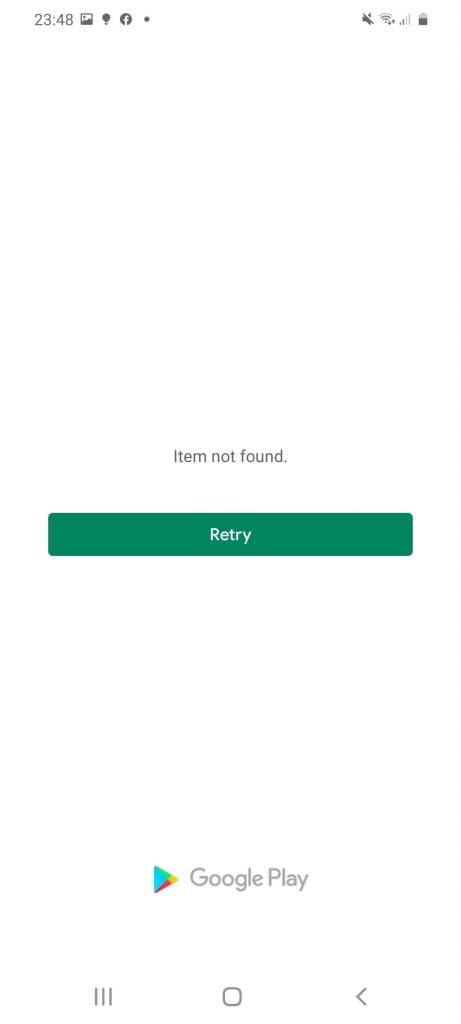This smartphone screenshot shows a device interface with various icons and notifications at the top. From left to right, the top row includes a time stamp showing 23:48, followed by a pictures icon, a light bulb icon, and a Facebook icon. To the far right, there is a sound icon indicating the sound is off, a Wi-Fi icon showing a strong connection, and a battery icon displaying approximately 50% charge.

The main content of the screenshot features a prominent error message in the center of the screen stating "Item not found." Below this message, there is a green button labeled "Retry." Further down, the Google Play logo is displayed along with the text "Google Play."

At the bottom of the screen, there are three primary navigation buttons: a "close all tabs" button, a home button, and a left-facing arrow, which is typically a back button. This screenshot appears to capture a failed search attempt on the Google Play Store, indicated by the error message "Item not found," and offers the user the option to retry the search using the "Retry" button.